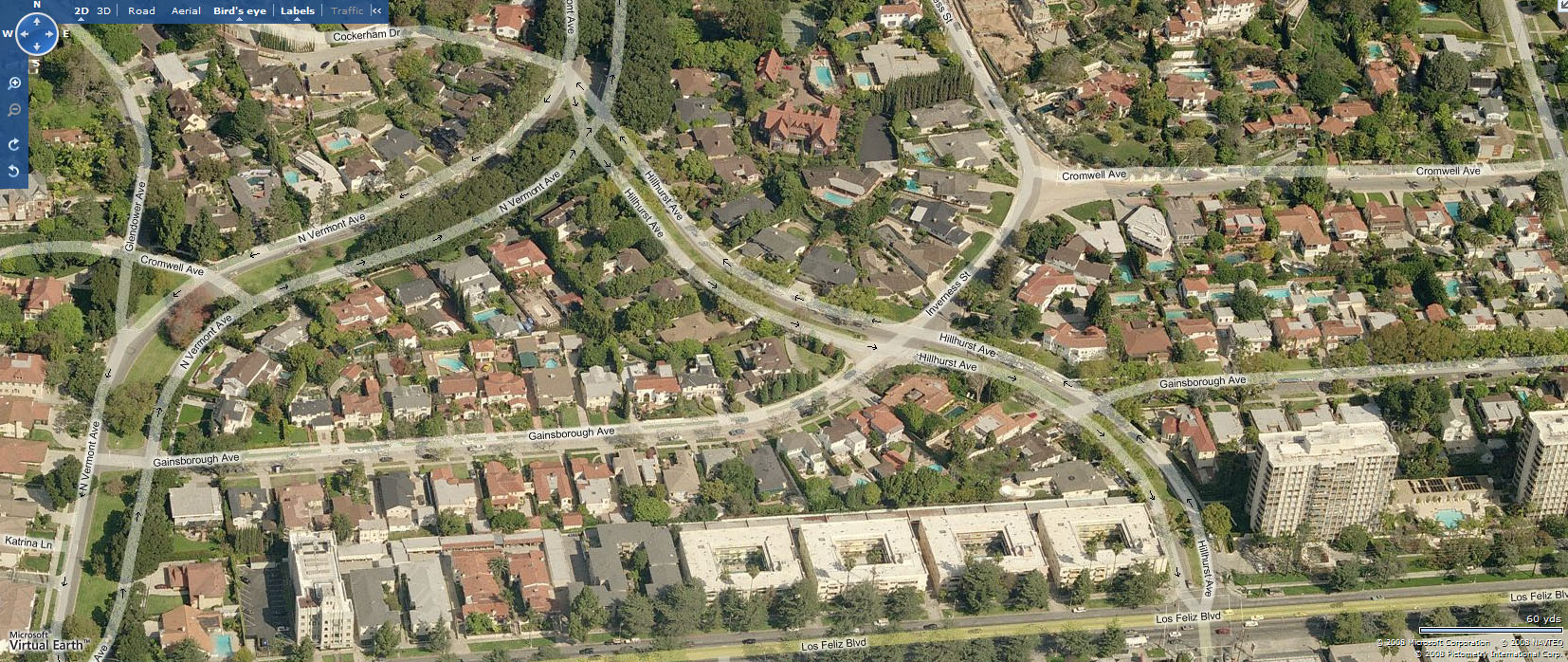An overhead image showing a detailed map of a subdivision. The perspective is slightly angled, with the view taken from above. Names of roads are clearly overlaid on the actual streets. The subdivision features numerous houses, many equipped with swimming pools, suggesting a warmer climate. There are a few apartment complexes situated at the bottom of the image, characterized by their square shape and central courtyards; there are four of these complexes. A main thoroughfare winds through the middle of the subdivision, dividing the image into two halves in a yin-yang pattern. In the upper left corner, detailed navigation symbols, including a compass indicating north, south, east, and west, are visible. A vertical bar on the left side, about one-quarter of the way down, features additional symbols, while the top right corner also includes symbols enclosed in a blue box. The layout highlights both the residential and communal aspects of the area.